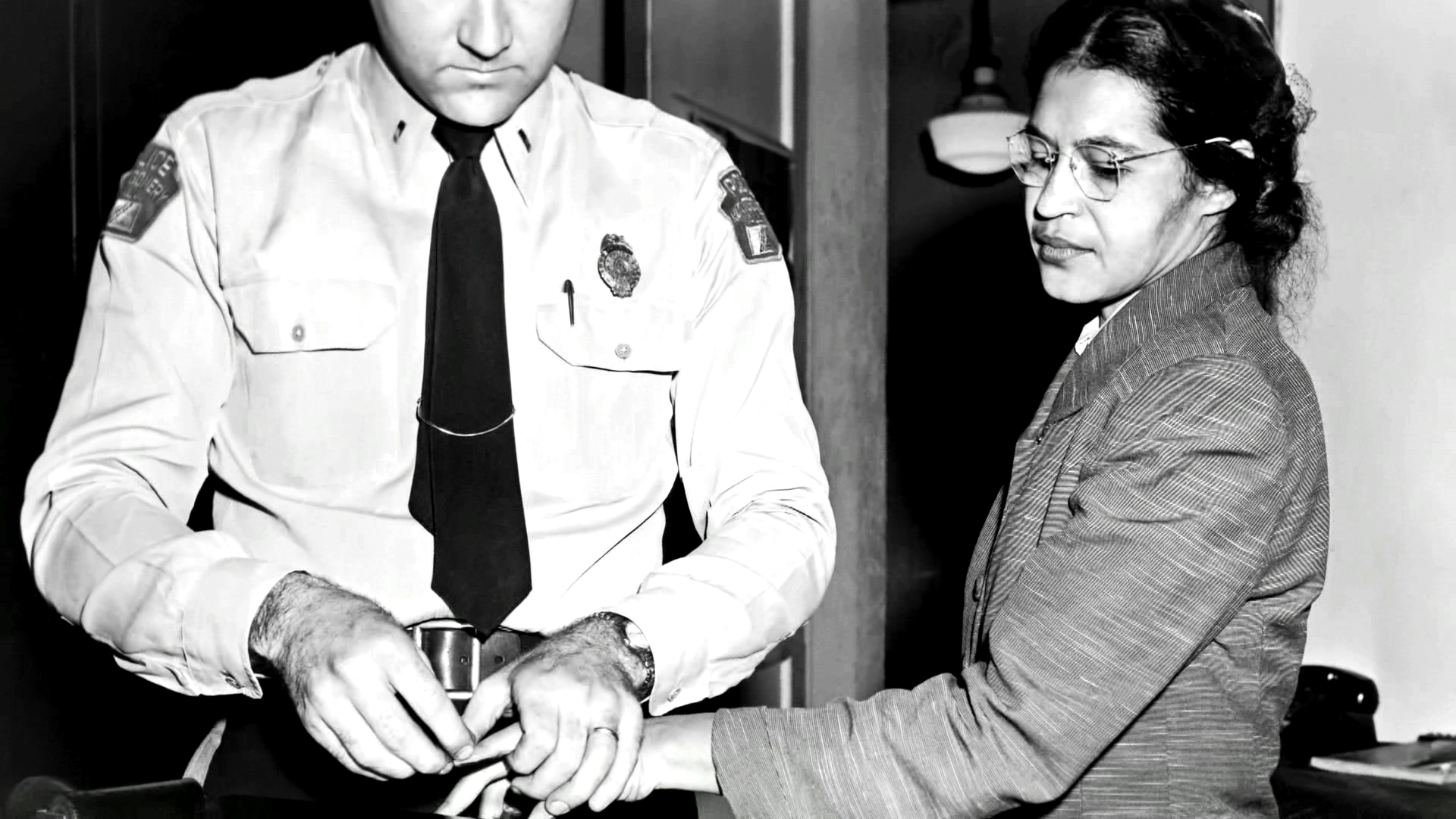In this horizontal, black-and-white photograph, a police officer is seen fingerprinting an individual who is likely Rosa Parks. The officer, whose face is visible only from the nose down, is dressed in a white button-down shirt with a tie, patches on each sleeve, a badge on his chest, a belt, and a gun at his side. His uniform includes a pen in his pocket, indicative of his official duties. The scene appears to occur in a plain, nondescript police room. The individual being fingerprinted, presumably Rosa Parks, has her black hair pulled back into a bun and wears white-rimmed glasses along with a grayish jacket. She is in a compliant posture, looking down at her hands as the officer holds her left hand to take fingerprints. An open door in the background adds a subtle context to the setting, emphasizing the procedural and solemn nature of this historical moment.